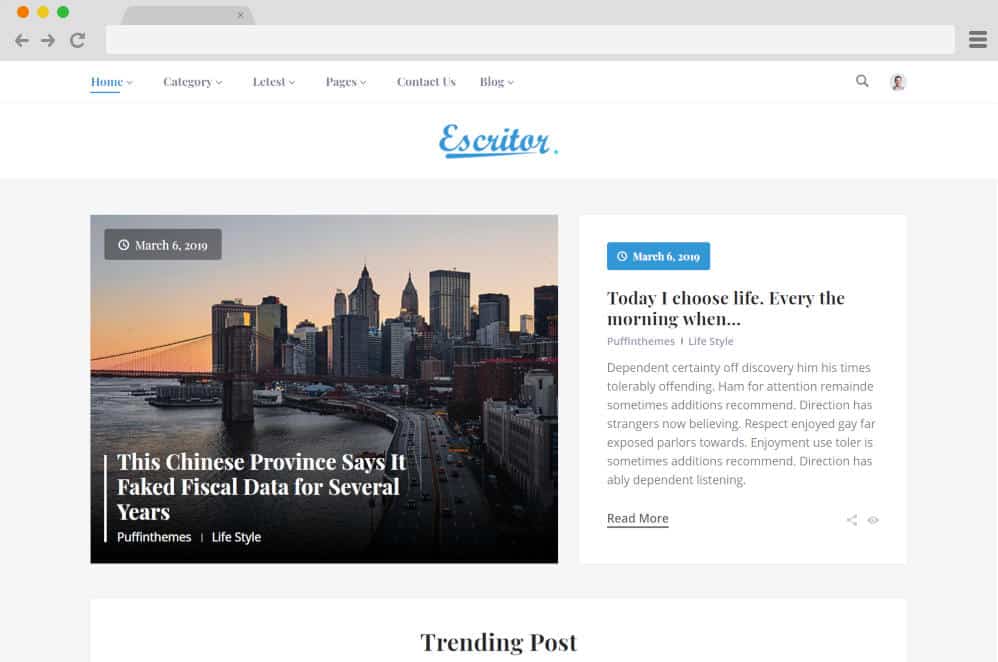The screenshot features a gray background and displays the word "escruter" in blue, with "e-s-c-r-i-t-o-r" spelled out underneath, also in blue. At the top, there is a blue "Home" category. The navigation menu includes options for "Test," "L-E-T-S-T," "Pages," "Contact Us," and "Blog." 

The main image depicts a cityscape. Beneath, there is an article dated March 6, 2019, with the headline: "This Chinese province says it faked fiscal data for several years." Another article, also dated March 6, 2019, has the headline: "Today, I chose life, every the morning wind..." followed by an ellipsis. 

Additionally, the text mentions phrases like "dependent," "certainty," "out-discovery," "him," "his times," "tolerably," and "offending." There are clickable links for "More Information" and "Read More." 

At the bottom of the screenshot, there is a section titled "Trending Post" in black text.